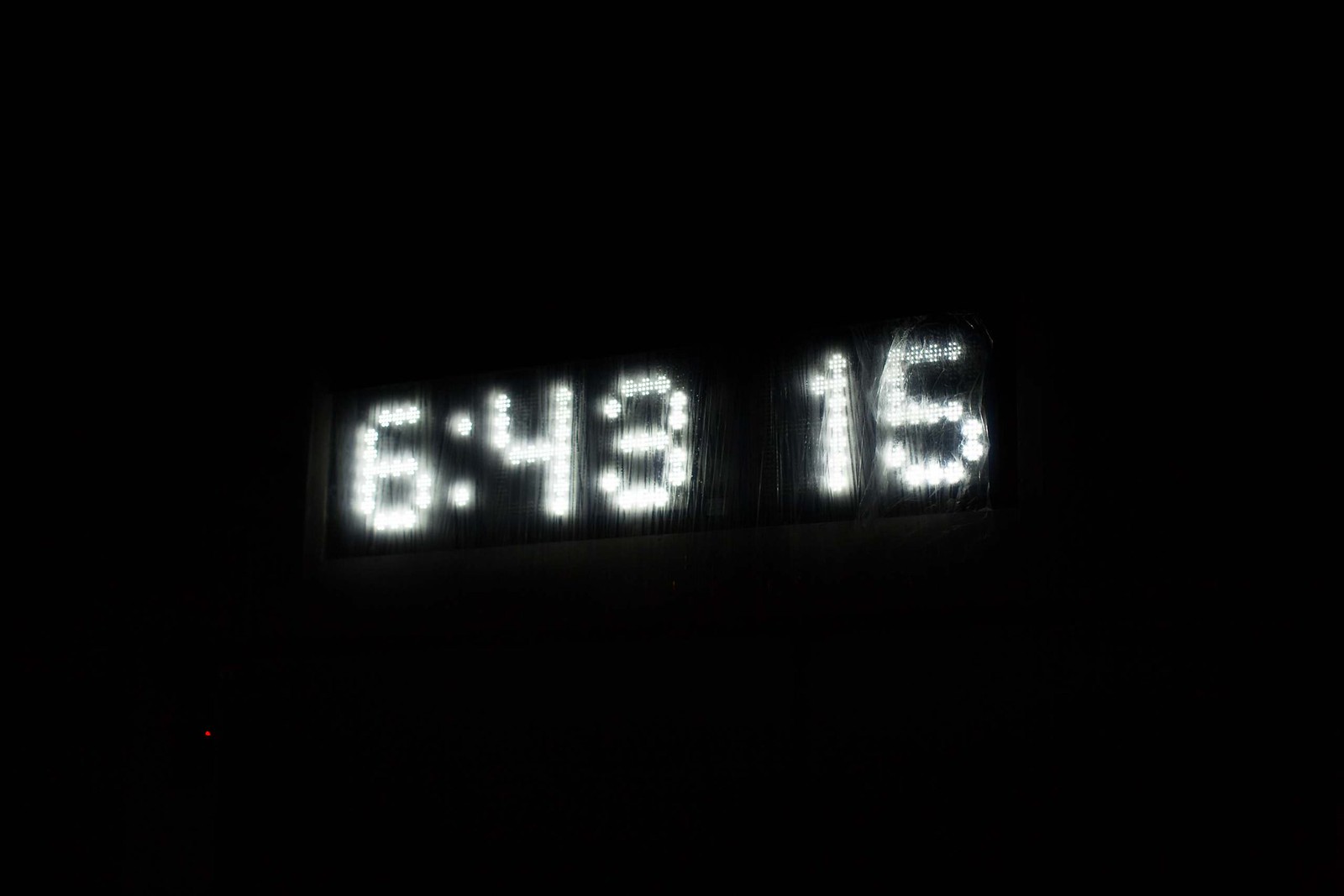In this rather blurry photograph, we see a digital clock displaying the time "6:43" followed by "15," likely representing seconds. The numbers are illuminated in white using a dotted digital printout, creating a bright contrast against a completely jet-black background. The image is taken in a dark setting, making the glowing numbers stand out even though they are slightly out of focus and appear somewhat angled. The individual dots that form the numbers are visible, with some dots on the "15" seeming dimmer than others. The absence of any distinguishing features or textures in the background makes it challenging to determine whether the clock is situated indoors or outdoors.